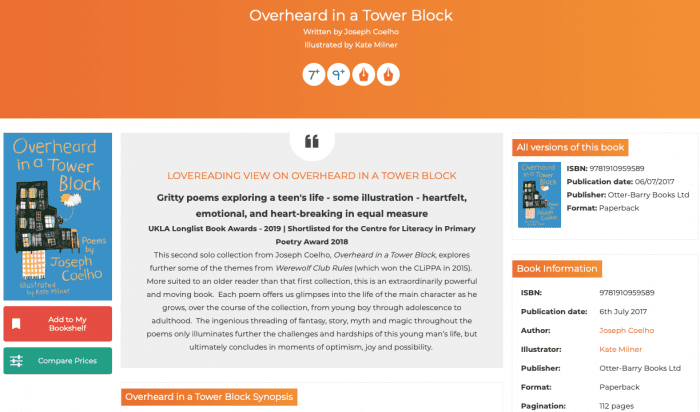The website features a book titled "Overheard in a Tower Block," authored by Joseph Coelho and illustrated by Kate Milner. Prominently displayed on the left side is an image of the book's cover, set against a blue background with a whimsical, almost childlike font. The cover illustration depicts a uniquely shaped bookcase, resembling a staircase, filled with various items, adding an intriguing visual element.

Below the book cover image, users can find interactive elements including a red button for an app and a green "Compare Prices" button.

Adjacent to the cover is a detailed description highlighting the book's content: "Groovy poems exploring a teen's life, accompanied by heartfelt and emotional illustrations that are heartbreaking in equal measure." This description seems to be part of a review, offering insight into the book’s appeal.

Furthermore, the page provides additional context, indicating that this is Joseph Coelho's second solo collection. It delves deeper into themes explored in his previous work, "Werewolf Club Rules," and is suggested to be more suitable for an older reader.

On the right side of the page, there is further book information, including the ISBN and publication date, ensuring potential buyers have all the necessary details at their fingertips.